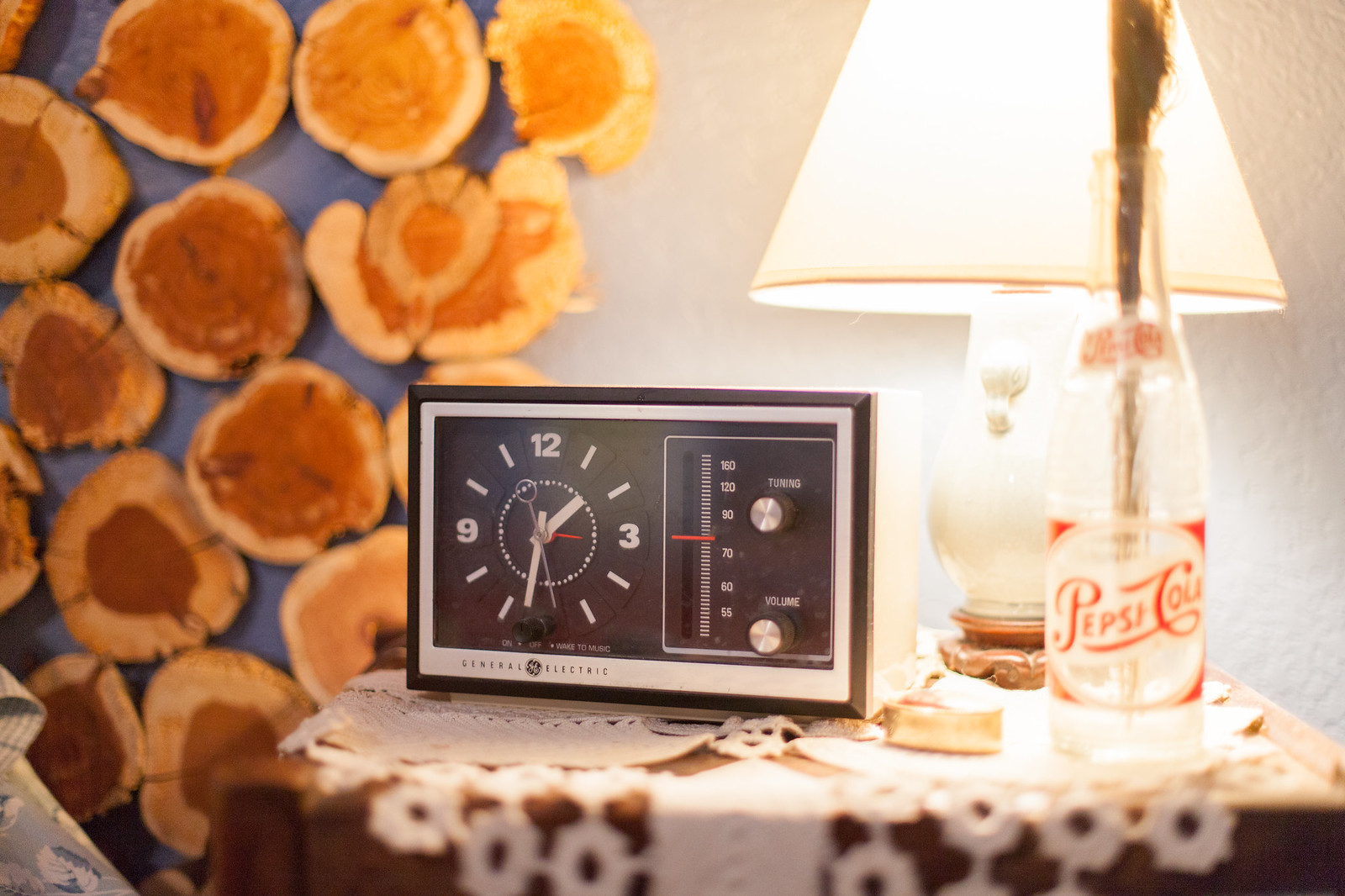The photograph showcases a rich, detailed interior scene centered around a wooden bedside table adorned with a white lace tablecloth. The focal point of the image is an old-fashioned General Electric alarm clock-radio, featuring a prominent black rectangular face with white numbers and clock hands, accompanied by dials for volume and tuning on its right side. Surrounding the clock-radio, on the right side is an iconic clear Pepsi Cola bottle with a red and white label that appears to be empty, containing a stick inside. A lit lamp with a white lampshade stands behind these items, casting a warm glow. The background reveals a plain white wall adorned with several round decorations, light brown on the outside with dark brown centers. This photograph, rendered in color, captures the blend of nostalgic and functional elements, possibly from a particular era, offering a snapshot that could easily serve for an interior design context.